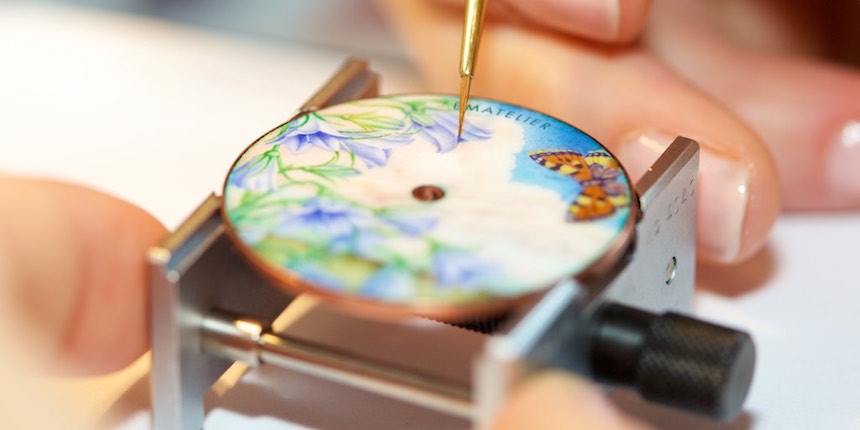This detailed, close-up image captures a small, intricately painted gold disk resting vertically atop a silver rectangular container. The container, akin to a vice, has no visible openings at the top and bottom and includes a black handle on the right side to adjust its grip. The disk, adorned with rich artwork, features vivid blue skies, white clouds, green vines, light purple flowers, and yellow and black butterflies. Two white hands, each gripping one side of the container, are delicately holding the setup, adding a sense of precision and care to the scene. A small, gold paintbrush extends from the top of the disk, appearing to add final touches to the purple flowers. The background is slightly blurred, highlighting the focused activity and emphasizing the intricate details of the artwork.